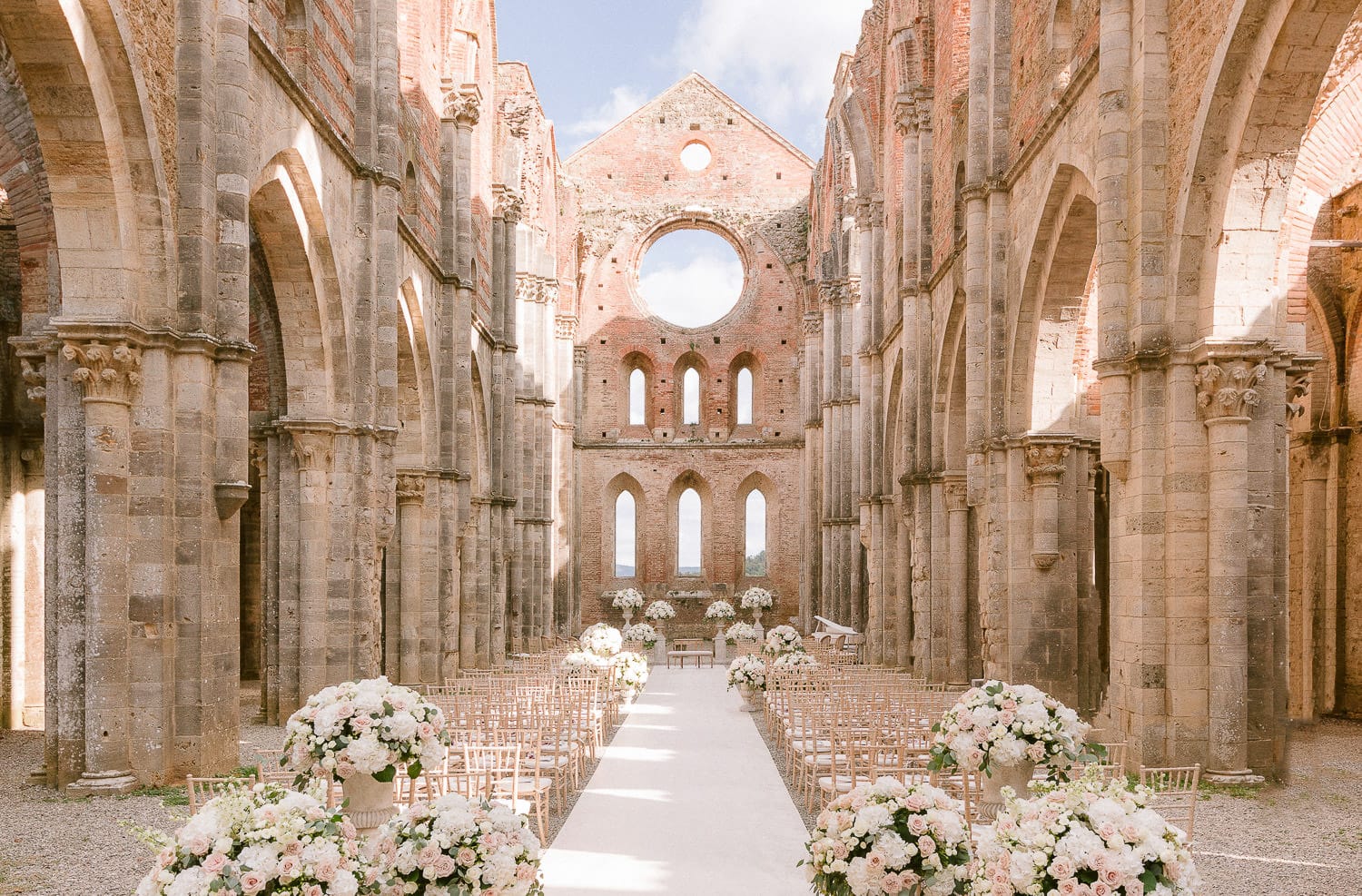This image captures the serene setup of an outdoor wedding venue resembling an open-air cathedral. The horizontally aligned picture features a stunning stone structure with walls, arches, and pillars shaded in brown or beige. The venue is devoid of people, emphasizing the meticulous preparations. In the foreground, a white carpet serving as the aisle runs down the center, flanked by rows of light wood chairs with white cushions. Abundant floral arrangements, blending white and light pink flowers in bouquets and small vases, grace both sides of the aisle and the altar area. The open-top stone structure allows a clear view of the blue sky adorned with white clouds, visible through a circular cutout in the triangular tip of the wall behind the altar. This setting, bathed in sunlight, harmonizes the rocky desert ground with the ethereal charm of white and pink flowers, making it a picturesque venue for the forthcoming wedding ceremony.